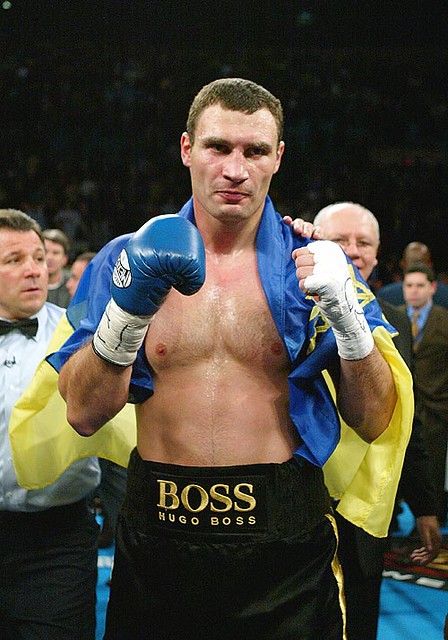This image captures a powerful moment featuring a prize fighter, whose identity is not immediately recalled but whose face is recognizable. The fighter is posed facing forward, shirtless, and exudes confidence and intensity. Draped over his neck and back is what appears to be a luxurious blue silk wrap. He is wearing black shorts with the word "Boss" prominently displayed in gold on the front, indicating they are Hugo Boss shorts. 

The fighter is pointing a blue boxing glove directly at the camera, creating a dynamic and engaging focal point. His left hand is bandaged, suggesting the glove has been recently removed. Part of a blue and yellow cape is visible below his elbows, with the blue fabric extending from his neck. 

In the background, to the left of the fighter, stands a referee dressed traditionally in a white shirt, dark pants, and a bow tie. Over the fighter's right shoulder, another man is seen with his right arm resting on the fighter's left shoulder, offering support. The fighter has short brown hair and an intense, fierce expression, capturing the essence of a warrior ready for battle.